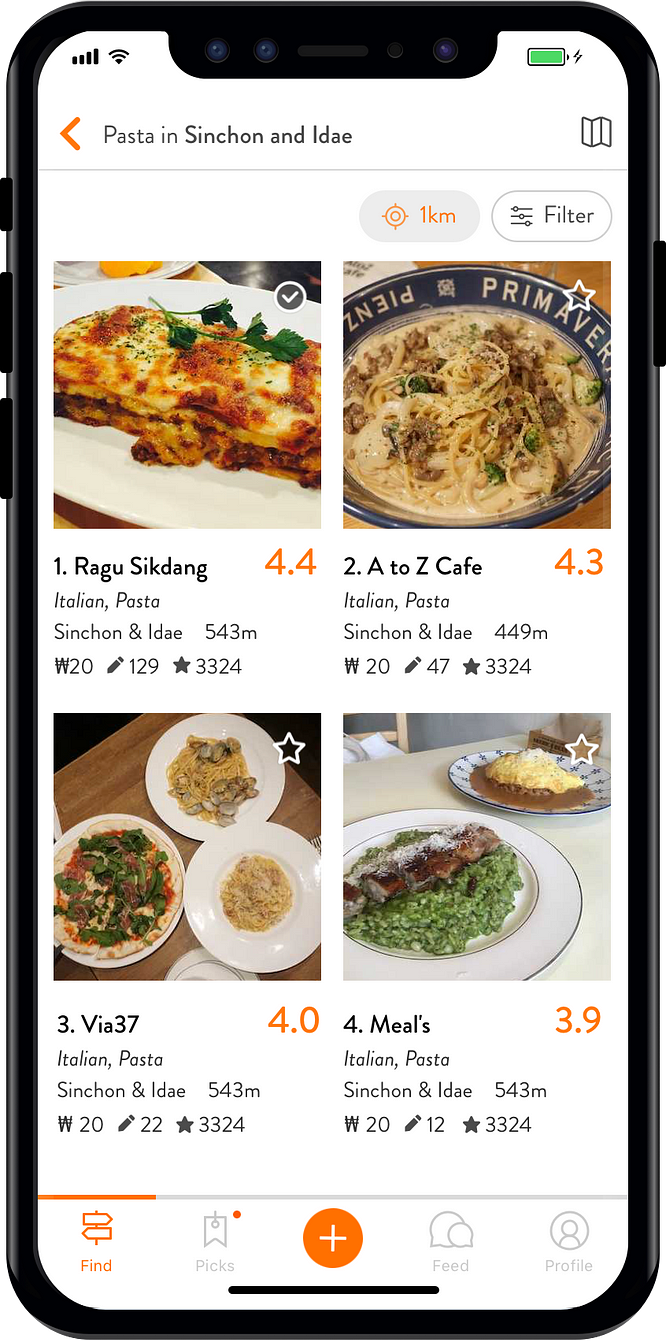This is a detailed smartphone screenshot of a meal recommendation website page. The page has a white background, and at the top, there are common status icons: a full green battery indicator and a Wi-Fi symbol. Below these icons, from left to right, are a left-facing orange arrow, the text "Pasta in Sinchon and Aidae," and a menu icon. Beneath this header, a text displays the distance as 1 kilometer and a filter button.

The main section of the page features four distinct images of plates of pasta, each accompanied by various details:

1. **Top Image:**
   - Restaurant: Rabu Sikdang
   - Rating: 4.4 stars
   - Cuisine: Italian pasta
   - Location: Sinchon and Aidae
   - Distance: 543 meters
   - Price: W20
   - User Reviews: 129 (represented by a pencil icon)
   - Total Reviews: 3,324

2. **Second Image (also a plate of pasta):**
   - Restaurant: A2Z Cafe
   - Rating: 4.3 stars
   - Cuisine: Italian pasta
   - Location: Sinchon and Aidae
   - Distance: 449 meters
   - Price: W20
   - User Reviews: 47
   - Total Reviews: 3,324

3. **Bottom Left Image:**
   - Description: Three plates of Italian pasta
   - Location: Sinchon and Aidae
   - Rating: 4.0 stars
   - Distance: 543 meters
   - Price: W20
   - User Reviews: 22
   - Total Reviews: 3,324

4. **Final Image:**
   - Description: Two plates
   - Category: Meals
   - Rating: 3.9 stars
   - Cuisine: Italian pasta
   - Location: Sinchon and Aidae
   - Distance: 543 meters
   - Price: W20
   - User Reviews: 12
   - Total Reviews: 3,324

At the very bottom of the screen, navigation icons are visible, labeled: "Find," "Pics," a central plus sign for adding content, "Feed," and "Profile Photo."

The overall page provides users with a detailed overview of various Italian pasta meals available within the Sinchon and Aidae area, rated and reviewed by other users.